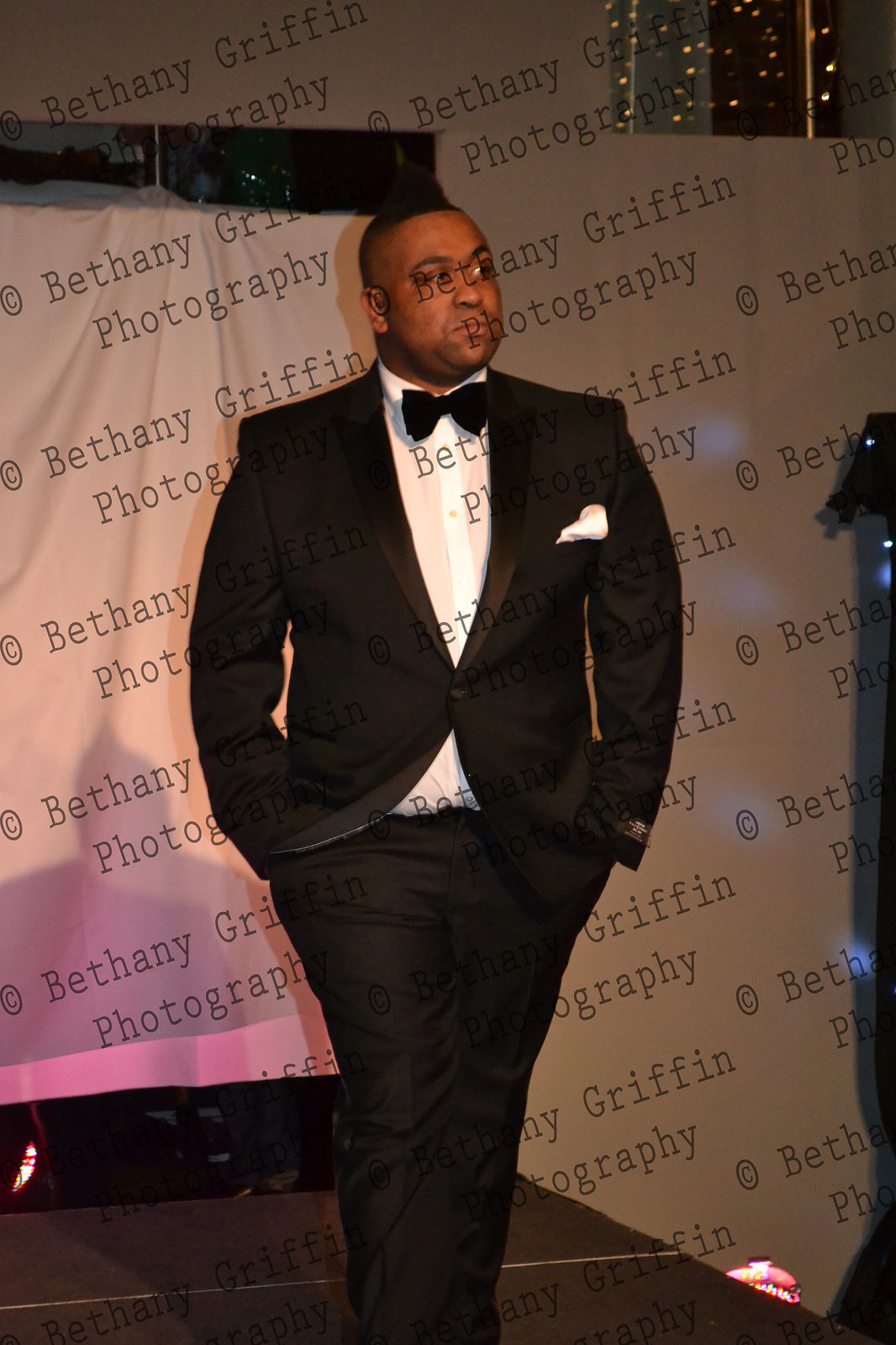The photograph captures a black man in his 30s, mid-walk, possibly on a runway or stage. He is dressed elegantly in a black tuxedo with a white button-down shirt and a black bow tie, and his hands are positioned in his pockets. His short black hair and stern expression give him a composed demeanor as he looks off to the right with his head slightly cocked. The background consists of stark white walls adorned with a continuous watermark reading "Bethany Griffin Photography" in black text, subtly angled across the image. The ground beneath him is black, reflecting his shadow, which shows a faint pinkish hue near the bottom of the wall. The overall positioning of the man is vertical and centrally aligned, suggesting a photoshoot or fashion event setting.